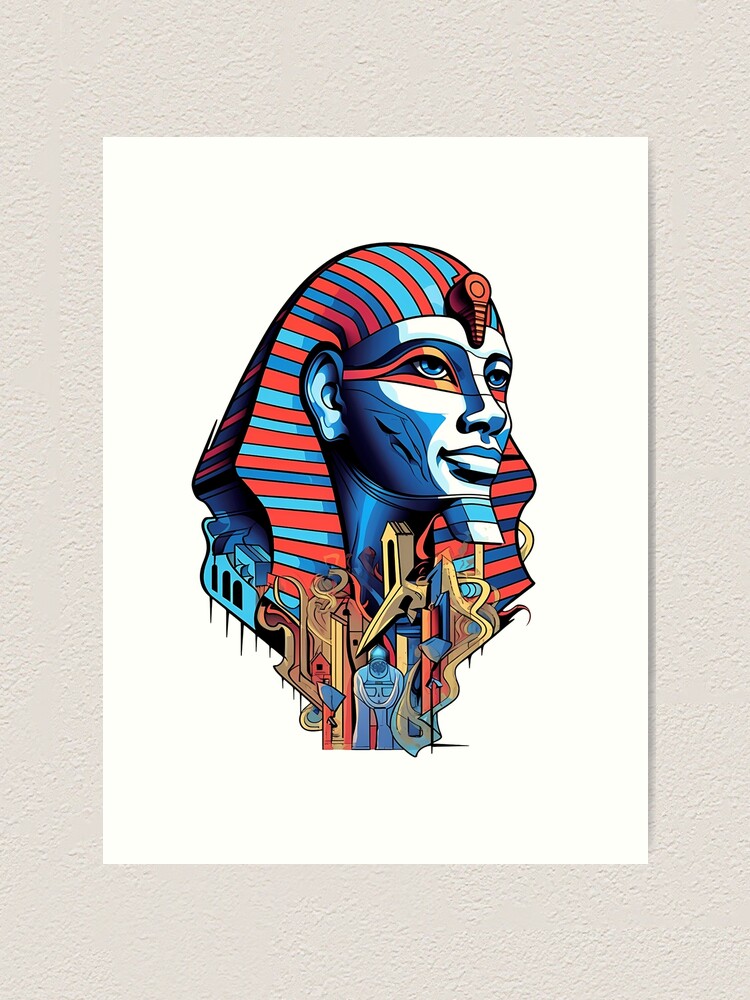The image depicted is a highly detailed and vibrant illustration of an Egyptian pharaoh or sphinx head, created on a solid white sheet of paper. This artwork, possibly a drawing or painting, is mounted against a white wall, providing a clear and brightly lit background that enhances its visibility. The pharaoh's face features a distinct blue tint, with orange and red mascara accentuating its eyes. The headdress adorning the pharaoh is intricately designed with blue and red stripes, while at its base, there are abstract orange and yellow structures intertwining with blue armor-like elements. The neck area below the headpiece showcases an elaborate abstract design, including a combination of light blue statues and golden yellow structures resembling roads and buildings, giving a sense of depth and significance to the illustration.